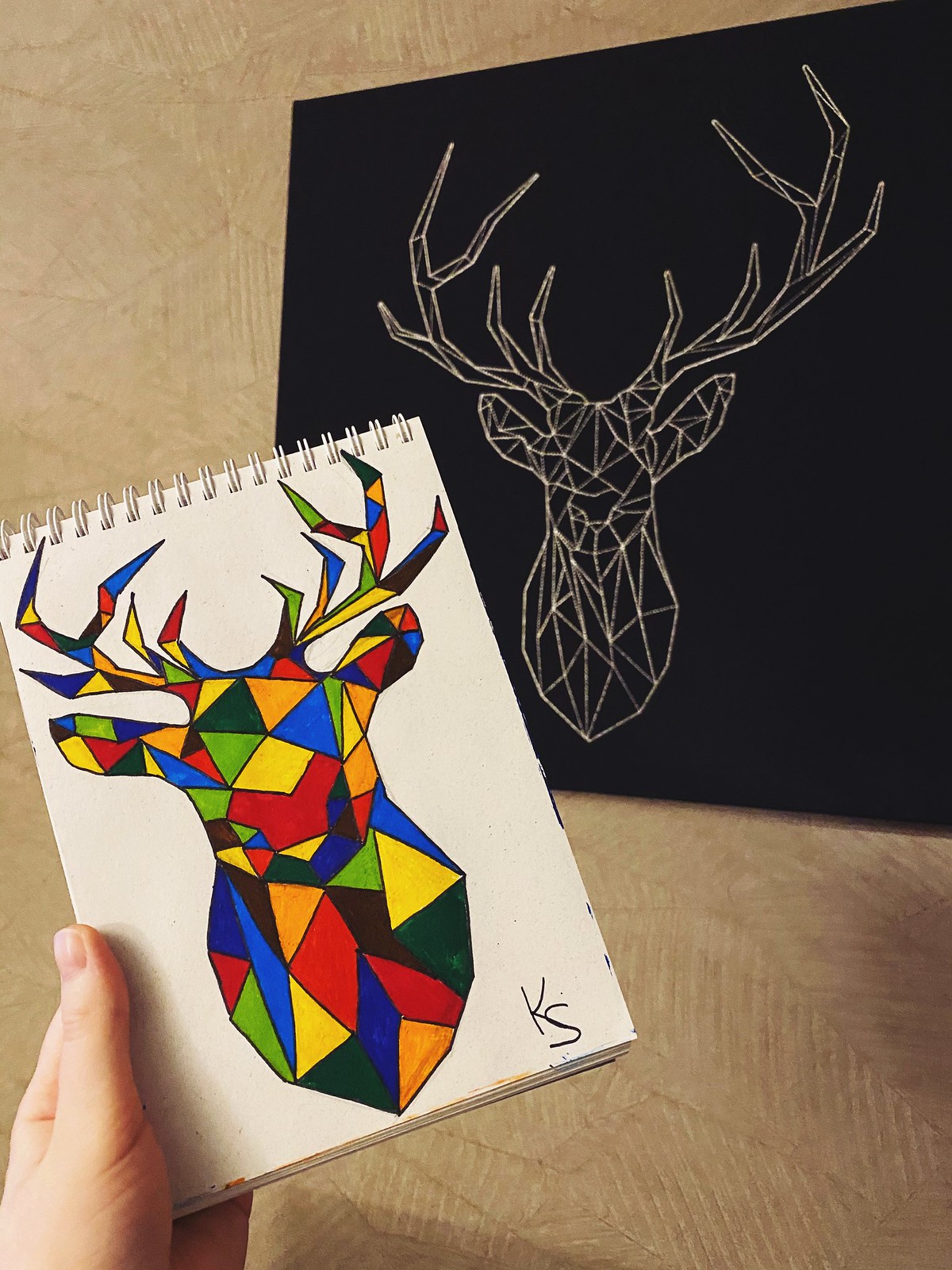The photograph is vertically oriented and taken from a slightly downward-facing angle, yet still providing a partial outward view, suggesting the photographer is holding an object in one hand while capturing the image with the other. The background reveals a textured, tan-colored surface, likely a couch cushion adorned with a subtle pattern of lines and shapes. A light source casts shadows across the cushion, enhancing the texture and depth of the background.

Central to the image is a black illustration of a deer, sketched with white lines that define its horns, neck, and body but noticeably lack details such as eyes. This illustration is mirrored on a sketchpad, which is held by a person's hand; the hand is positioned in the lower portion of the frame. The depicted sketch on the pad features the same deer figure, reinterpreted into various geometric shapes, all carefully colored. The bottom of the sketchpad displays the letters "KS," likely indicating either the initials of the artist or a signature.